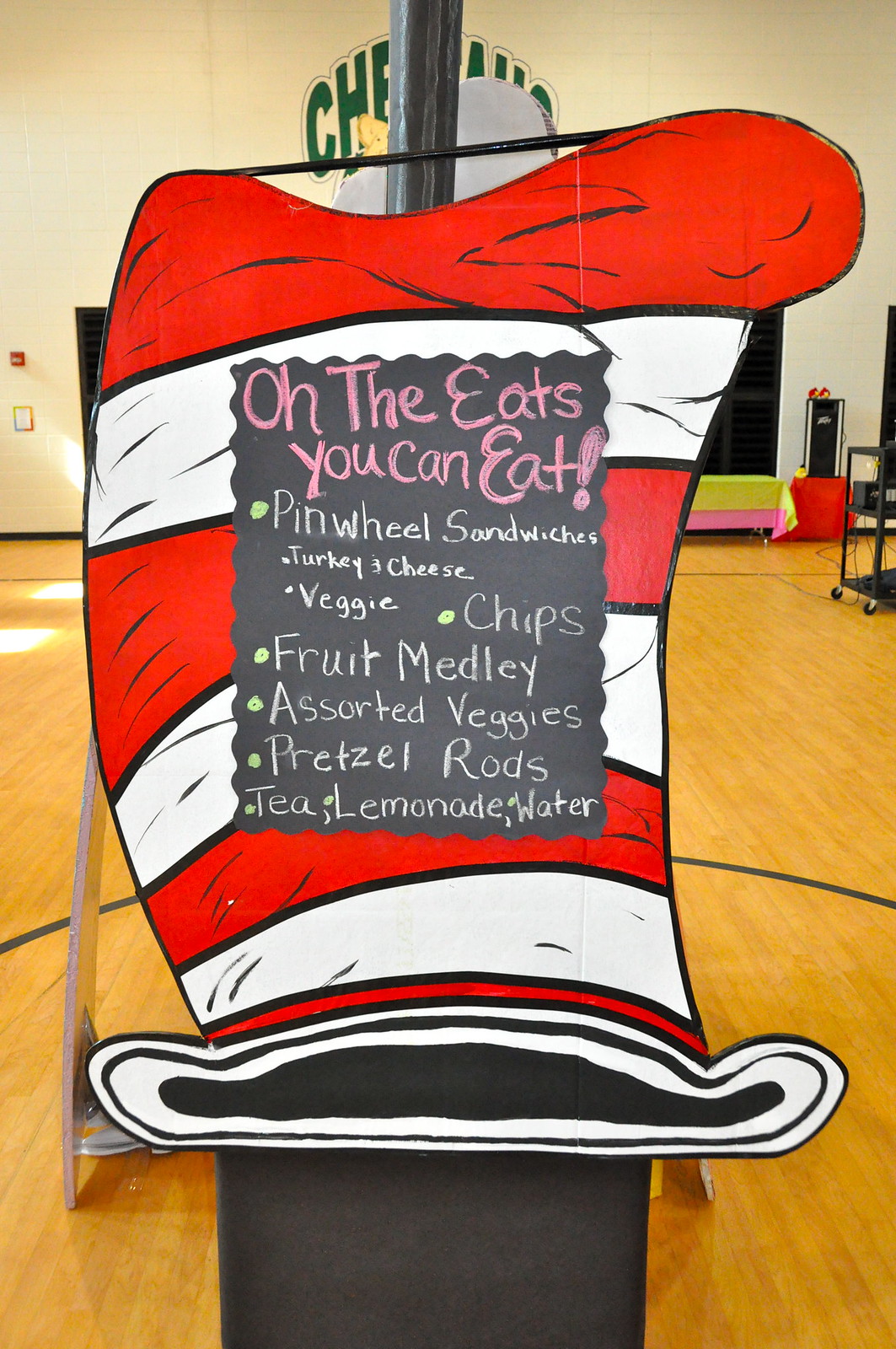This image shows a scene inside a gymnasium, indicated by the light brown wooden or vinyl floor with lines and a partial logo that reads "CHE." At the center of the photo, there's a distinctive, tall vertical sign resembling Dr. Seuss's iconic red and white striped hat. This hat features a black chalkboard area in the middle with festive pink chalk writing at the top that says, "Oh, the eats you can eat." Below this heading, detailed in yellow bullet points with white text, a menu lists pinwheel sandwiches (including turkey and cheese, and veggie options), chips, fruit medley, assorted veggies, pretzel rods, tea, lemonade, and water. The sign appears to be attached to a metal bar at the top. In the blurred background, you can see a white wall marked by green writings obscured by a pole, along with a cart typically used for a TV and a speaker, suggesting that this setting is prepared for an event, possibly child-oriented given the playful menu and theme.